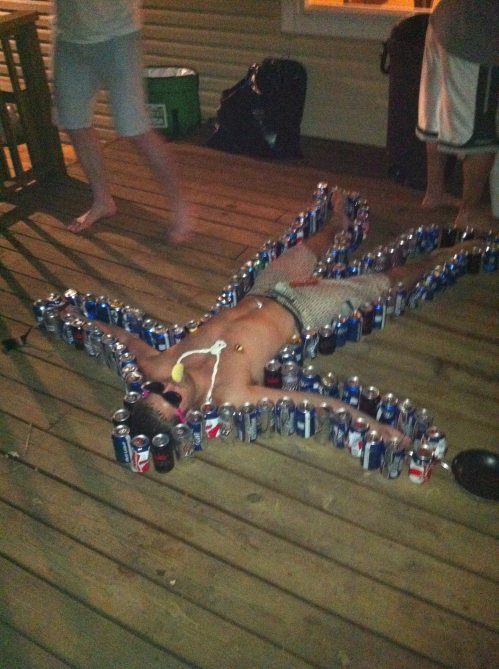The image captures a nighttime outdoor frat party scene on a wooden deck. In the center lies a shirtless, Caucasian man with short brown hair and black sunglasses, sprawled on his back with his arms and legs wide open. He is outlined by an assortment of beer cans in varied colors - blue, black, and white - arranged meticulously around his body, reminiscent of a police chalk drawing. A straw extends from his mouth to one of the beer cans, indicating he’s drinking from it. He is wearing light tan shorts. In the background, we see the lower halves of two other individuals. One, on the left side of the image, is wearing a white shirt and grayish shorts, while the other, on the right, dons black and white basketball shorts with a gray shirt. Both are barefoot. Scattered trash is visible on the wooden deck floor, contributing to the party atmosphere.